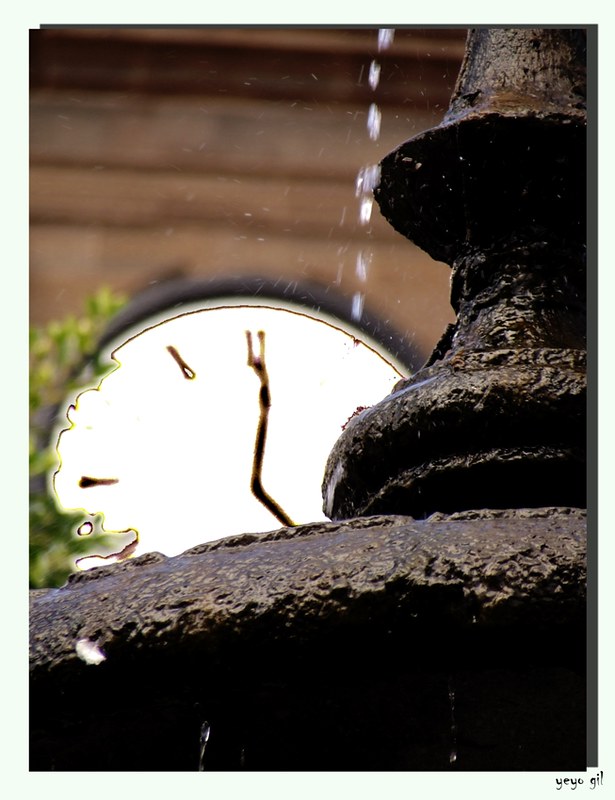This close-up photograph captures a detailed section of an outdoor iron water fountain, which features a large, dark brown to black base. The fountain rises into a series of triangular sections, with the topmost portion resembling a pointed hat. Water droplets, or possibly light reflections, can be seen falling from the structure, appearing somewhat blurred. Beneath this, a half-circle shape suggests the outline of a clock, although no specific clock details are visible. The background is slightly out of focus but reveals the wall of a house, appearing brown, and a mix of green plant life surrounding the fountain. Additionally, there is a white circular object resembling a clock face near the bottom of the image, enhancing the overall scene's distinctive, rustic charm.